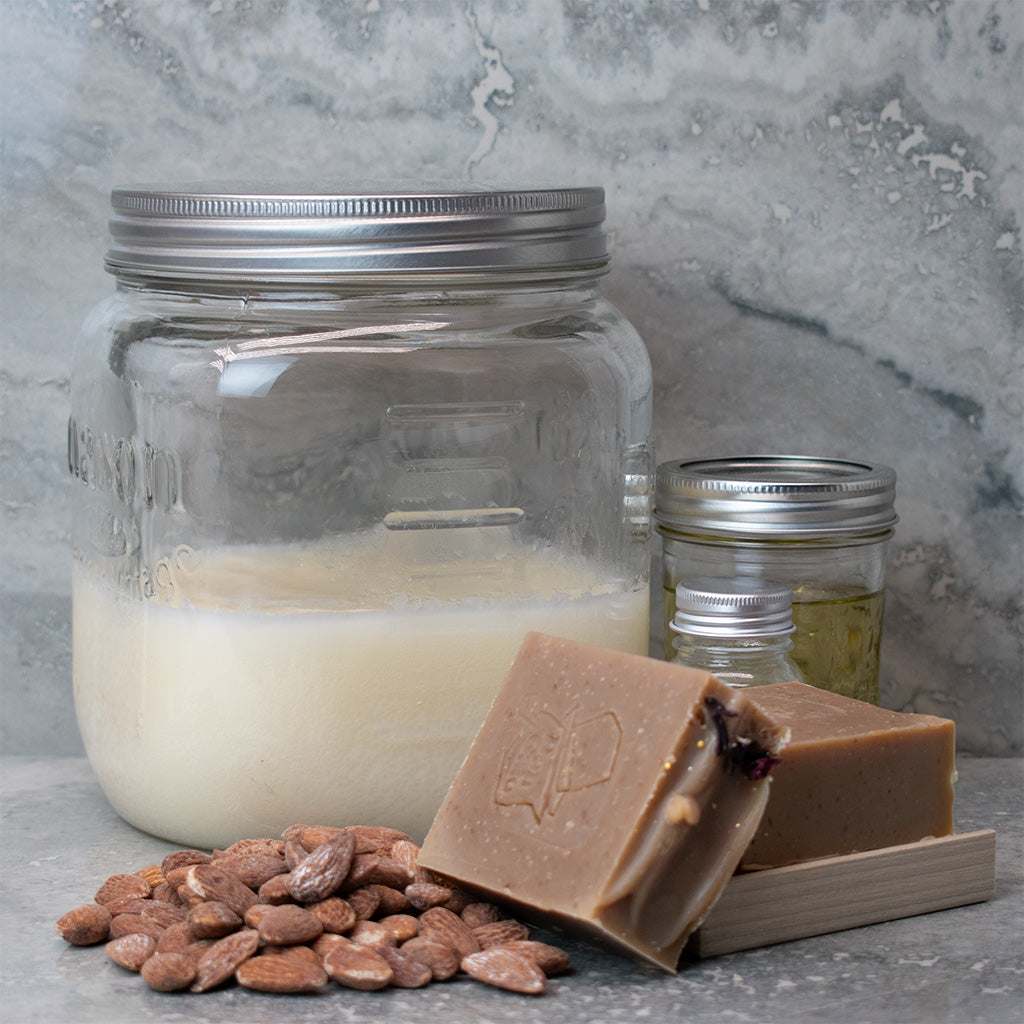The square photograph captures a detailed view of a gray granite countertop with white flecks, accompanied by a backdrop of matching gray granite featuring prominent black and white veining. In the lower left corner, a handful of roasted whole almonds are scattered across the countertop. Directly to the right of the almonds are two perfectly square chunks of what appears to be fudge, with one piece lying flat and the other leaning against it. Behind these treats stands a large mason jar with a silver lid, filled halfway with a white substance. Adjacent to this sizable jar is a smaller mason jar, also with a silver top. In front of the smaller mason jar, the top of a glass bottle with a silver screw-on cap is visible, although the rest of the bottle remains out of frame.